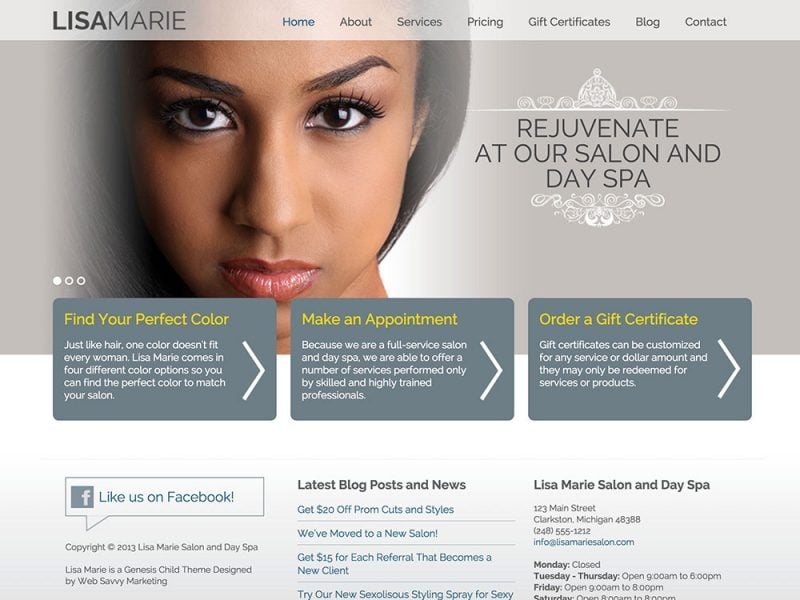The image depicts a detailed and visually striking website interface designed for a beauty salon and day spa. Dominating the scene is a large, square background featuring a close-up image of an African-American woman. The framing focuses on her face from the chin upward, highlighting her elegantly applied makeup, including lipstick, mascara, false lashes, and both top and bottom eyeliner. Her dark, long hair cascades around her, and she’s gazing intently at the camera.

At the top of the image, the name "Lisa Marie" is prominently displayed. The navigation menu overlays her forehead area, listing options such as Home, About, Services, Pricing, Gift Certificates, Blog, and Contact, with the Home option highlighted in blue.

To the right of the page, there is a small crown icon, beneath which the tagline "Rejuvenate at our Salon and Day Spa" is written, accompanied by another small white icon below it. 

Below this section, the webpage offers interactive features. There are three circular indicators suggesting additional images can be viewed by scrolling. A highlighted yellow text reads "Find Your Perfect Color," followed by a brief description. Next to this, a grey box with yellow text prompts users to "Make an Appointment," and includes another descriptive blurb. The third grey box invites users to "Order a Gift Certificate," with a similar accompanying blurb and a white arrow indicating further navigation options.

The bottom section of the image includes several additional interactive elements: a prompt to like the business on Facebook, a copyright notice, and access to the latest blog posts and news. There are links detailing various promotions, happenings, and referral information. Finally, the website provides the salon's address, hours of operation, and contact details at the bottom right corner.